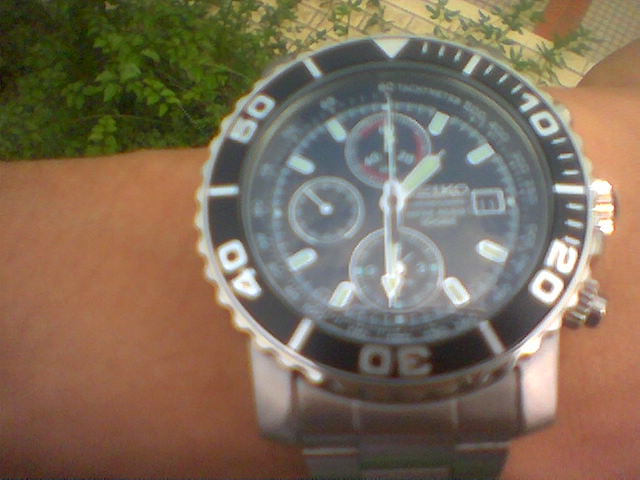The image showcases a close-up of a Seiko analog wristwatch, prominently featuring a silver stretch band worn by an arm with an ambiguous gender. The watch boasts a thick, silver exterior and a black bezel with indented markings indicating 10, 20, 30, 40, 50, akin to those found on a diver's watch, possibly used for timing. At the center, the brand name "Seiko" is inscribed, and it includes additional features such as three sub-dials, potential moon phases, temperature, and altimeter indicators. The watch hands are neon and designed to glow in the dark. The background consists of greenery, including what appears to be a bush or tree, possibly jasmine or lemon, along with tile surfaces, suggesting the photo was taken outdoors. The image is somewhat blurry, emphasizing the overall intricate design and multifaceted functionalities of the wristwatch.